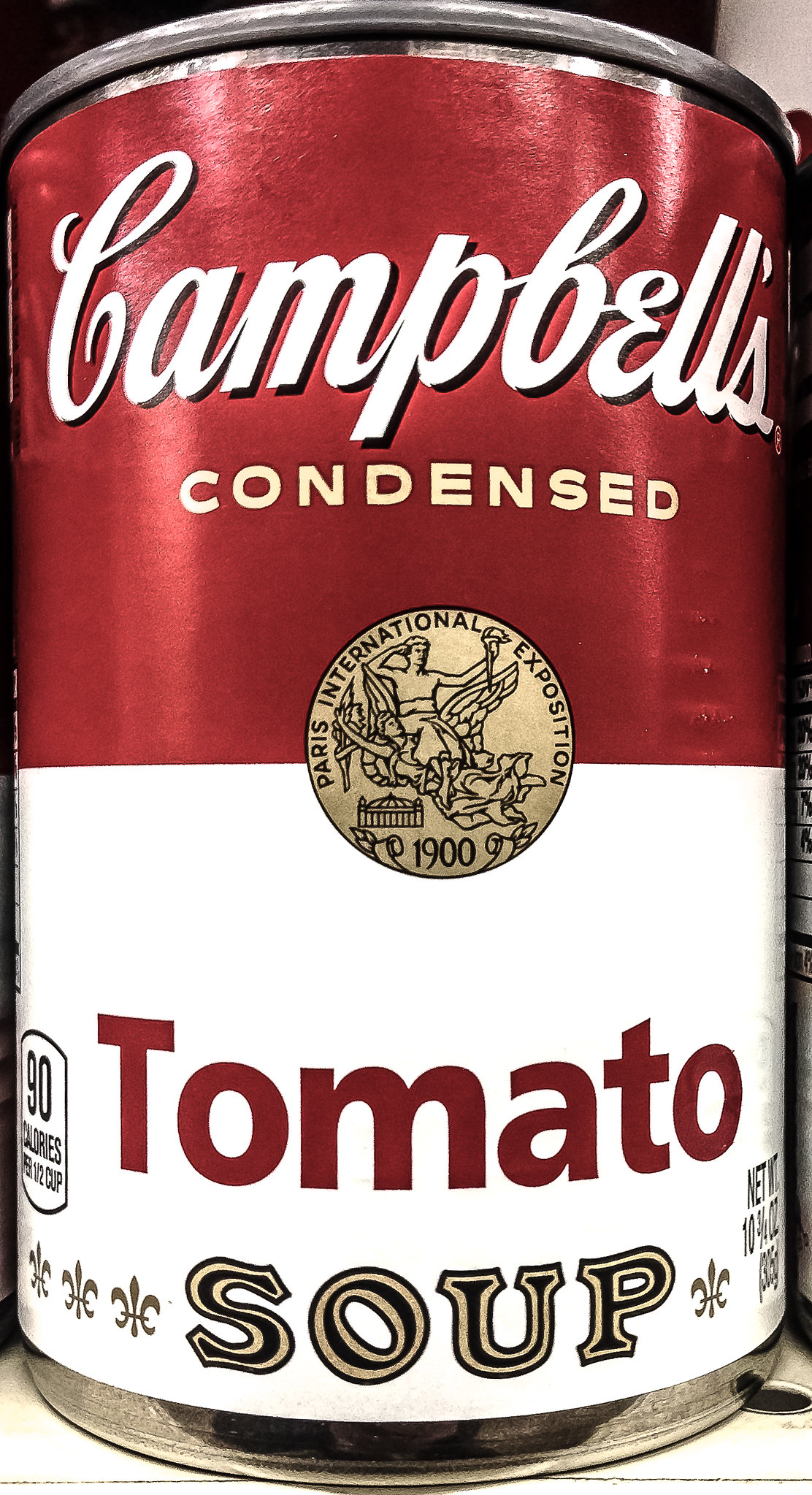This close-up, portrait-oriented photograph captures a can of Campbell's Condensed Tomato Soup in sharp detail. The cylindrical tin rounds off slightly at both the top and bottom, enhancing the viewer's focus on the familiar design. The can's top is metallic aluminum, distinct against the vibrant label below it. The upper half of the label is adorned in Campbell's iconic red, featuring their signature script "Campbell's" in white, with "Condensed" elegantly printed in gold lettering beneath it. Centrally positioned, bridging the red upper and white lower halves of the label, is the Paris International Exposition 1900 stamp, adding a touch of historical prestige. Lower on the left side of the label, the nutritional information is noted, including the fact that the soup contains 90 calories. Adjacent to this, the net weight of the product is clearly marked, completing the quintessential look of this beloved pantry staple.